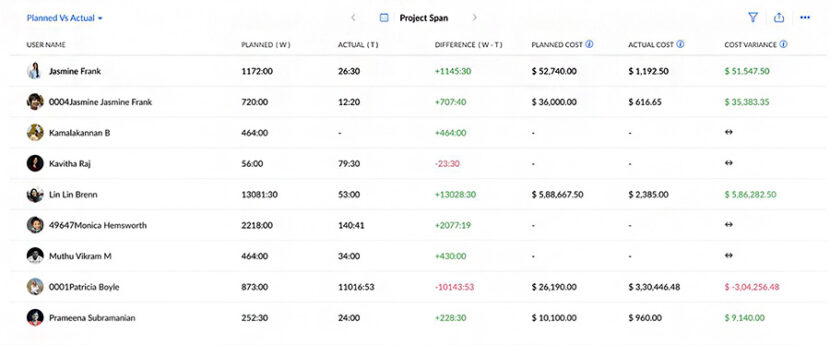The image displays a detailed table comparing planned versus actual metrics for a list of individuals. The table is set against a white background. 

In the top left corner, a blue header reads "Planned vs. Actual." Beneath it, the table is divided into multiple columns, specifically: 'Username,' 'Planned Time (W),' 'Actual Time (T),' 'Difference (W - T),' 'Planned Cost,' 'Actual Cost,' and 'Cost Variance.'

**Column Details:**
1. **Username:**
   - Each username is paired with an icon avatar. Below are the usernames in order:
     1. Jasmine Frank
     2. 0004 Jasmine
     3. Jasmine Frank
     4. Kamalakanon B
     5. Kavitha Raj
     6. Linlin Brin
     7. 49647 Monica Hemsworth
     8. Muthu Vikram M
     9. 0001 Patricia Boyle
     10. Pramina Subramanian

2. **Planned Time (W):**
   - The planned time entries are as follows:
     1. 1172:00
     2. 720.00
     3. 464.00
     4. 56:00
     5. 13081:30
     6. 2218:00
     7. 464.00
     8. 873.00
     9. 252:30

3. **Actual Time (T):**
   - The actual time entries are:
     1. 26:30
     2. 12:20
     3. -
     4. 79:30
     5. 53.00
     6. 140:41
     7. 34:00
     8. 11016:53
     9. 24:00

4. **Difference (W - T):**
   - The difference between planned and actual times, with red indicating negative values and green indicating positive values, are:
     1. 1145:30
     2. +707:40
     3. +464:00
     4. -23:30
     5. +13028:30
     6. +2077:19
     7. +430:00
     8. -10143:53
     9. +228:30

5. **Planned Cost:**
   - Planned costs, noted in dollars, are:
     1. $52,740
     2. $36,000
     3. -
     4. -
     5. $5,88,667.50
     6. -
     7. -
     8. $26,190
     9. $10,100

6. **Actual Cost:**
   - Actual costs, also in dollars, are:
     1. $1,192.50
     2. $616.65
     3. -
     4. -
     5. $2,385,000
     6. -
     7. -
     8. $3,304,256.48
     9. $9,600

7. **Cost Variance:**
   - A comparison of planned versus actual costs, denoted with green for positive variances and red for negative variances, is as follows:
     1. $51,547
     2. $35,038,300.35
     3. -
     4. -
     5. $5,086,282.50
     6. -
     7. -
     8. $-3,304,256.48
     9. $9,140

The table succinctly lays out a comprehensive comparison of planned versus actual metrics in both time and cost for each listed individual, with clear visual indicators for variances.